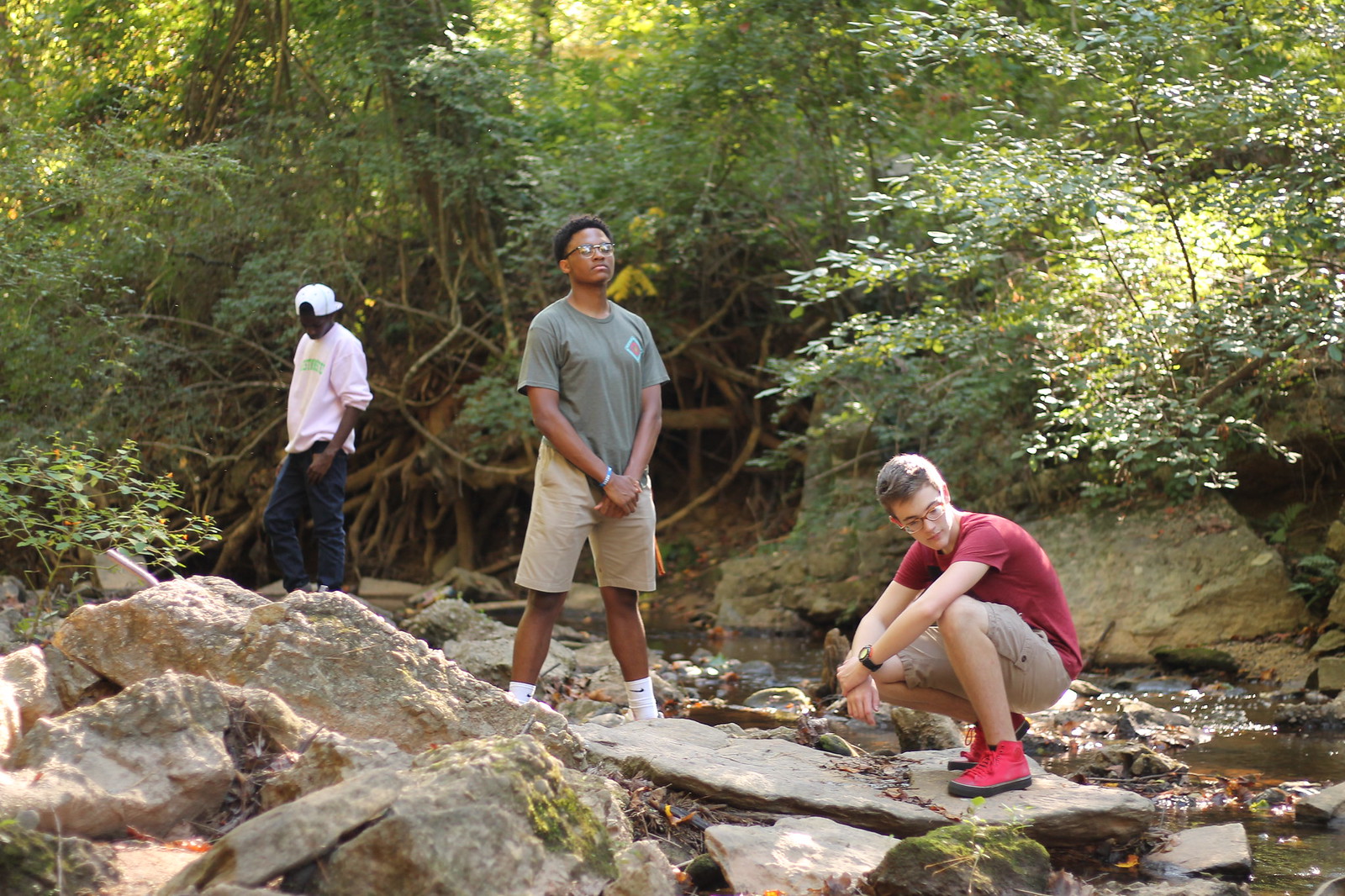The photograph captures a picturesque outdoor scene featuring three teenagers posing by a small creek. The background is dominated by a dense tree line of thick shrubbery and trees, which form a natural barrier that obscures the view beyond and creates a lush backdrop. In the foreground, a large gray boulder with patches of moss and vegetation sits prominently in the bottom left corner. The creek itself is filled with rocks and has light, green-tinged water gently flowing through it.

At the center of the image, three people are arranged on the rocky surface near the creek. On the left, a black teenager wearing blue jeans, a long-sleeve pink shirt, and a white baseball cap turned backward is looking downward. In the middle, another black teenager, dressed in khaki shorts and a green t-shirt with high white socks, stands with his hands crossed near his groin area. To the right, a white teenager is crouched down, wearing a red short-sleeve shirt, khaki shorts, red shoes, and a black watch.

The colors in the photograph are a mix of natural tones and vivid clothing hues, including shades of gray, green, red, blue, and brown. The setting appears to be a tranquil outdoor location, likely captured in the middle of the day, with the trio centered amidst the rocky stream and vibrant greenery.